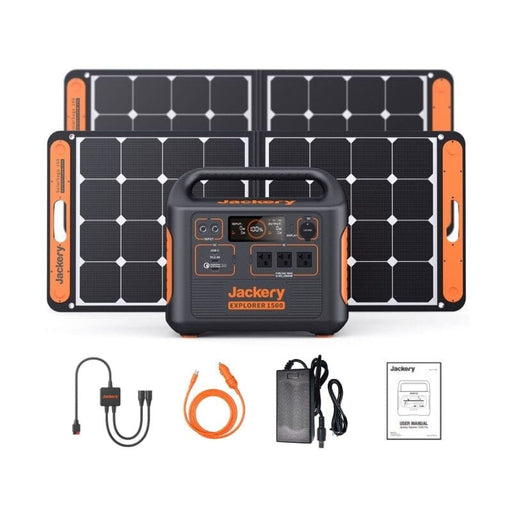The image displays a Jackery Explorer 1500 portable power station along with its accessories, set against a white background. The main unit is a black or dark charcoal gray rectangular box with rounded edges and orange accents, including a large handle and orange buttons. The front of the power station features multiple outlets and ports, including three three-prong AC outlets. The unit prominently displays the name "Jackery Explorer 1500" in orange lettering. 

Behind the power station are two foldable solar panel units, each comprised of two connected panels forming a four-by-four grid of black photovoltaic cells, bordered with orange handles that allow them to be carried like briefcases. The solar panels can be extended outwards or folded inward for easy transport.

At the bottom of the image, a selection of cables and accessories are displayed. These include a black USB adapter, an orange car charging cable, an AC wall adapter, and a black power supply brick. Accompanying these items is a white instruction manual that also bears the Jackery logo. This setup suggests the product is designed for off-grid power solutions, suitable for camping or emergency backup, with the solar panels providing renewable energy to charge the battery station.